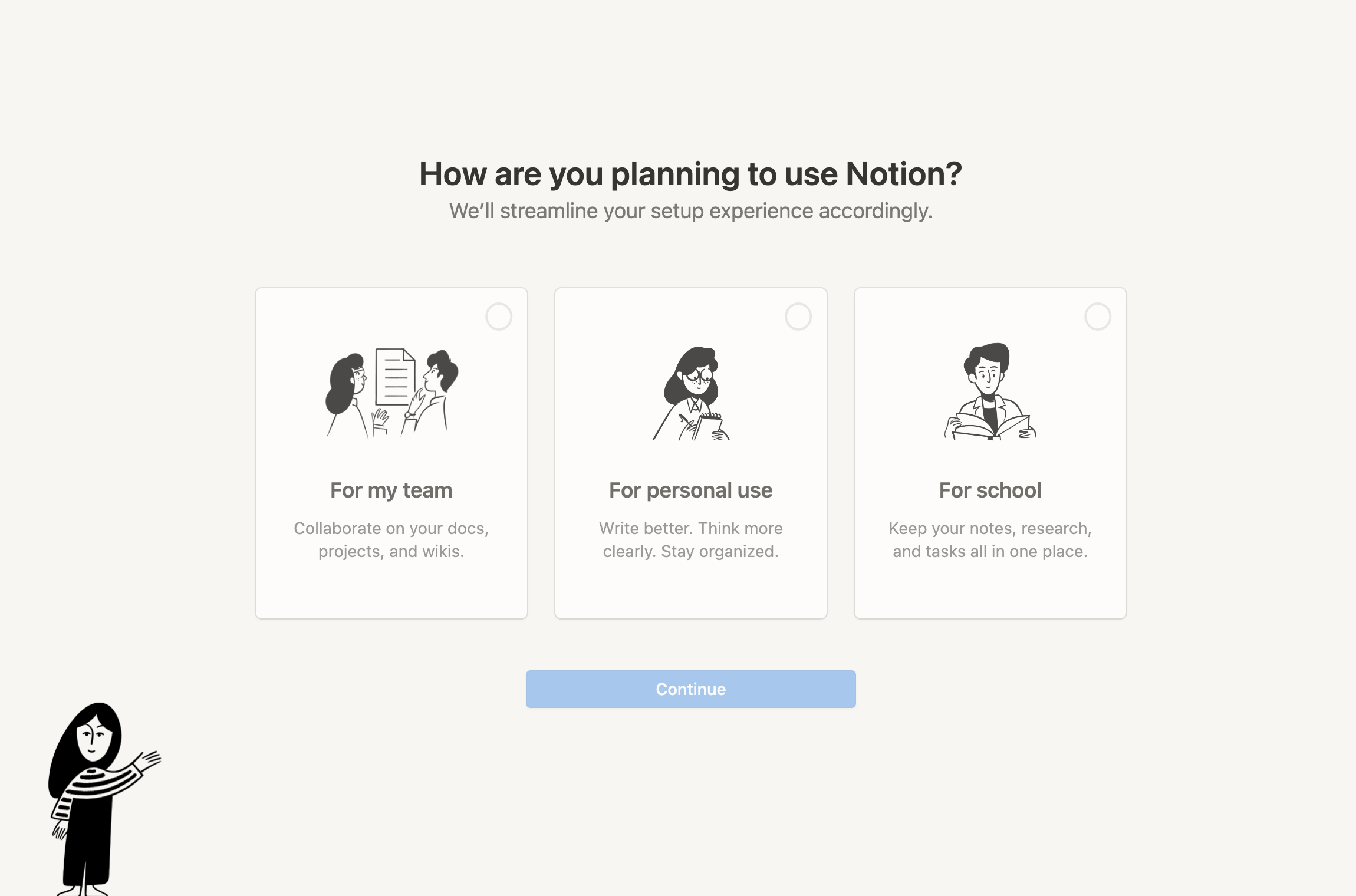The image displays a light gray rectangular screen with a centered header in bold, black text that reads, "How are you planning to use Notion?" Beneath this header, in smaller, gray, non-bold text, it says, "We'll streamline your setup experience accordingly." Below this, there are three distinct white rectangles with gray borders, each featuring a clickable circle icon in the top right corner to select an option.

The first rectangle shows an illustration of two cartoon characters examining a picture or document on the wall. The bold heading beneath this illustration reads, "For my team," and the accompanying text in smaller, non-bold font says, "Collaborate on your docs, projects, and wikis."

The second rectangle features a cartoon woman writing in a notepad. Its bold heading states, "For personal use," with the smaller text underneath saying, "Write better, think more clearly, stay organized."

The third rectangle depicts a cartoon man reading a book. The bold heading here is "For school," and the smaller text below reads, "Keep your notes, research, and tasks all in one place."

Under these options is a long, thin rectangular button in light blue, which says "Continue" in white text. This button is presumed to turn darker blue upon selecting an option, but none of the tick boxes are currently selected, keeping it light blue.

Towards the bottom left of the screen, there is an additional cartoon illustration of a woman with long, dark hair, wearing a striped shirt or shawl and black pants.